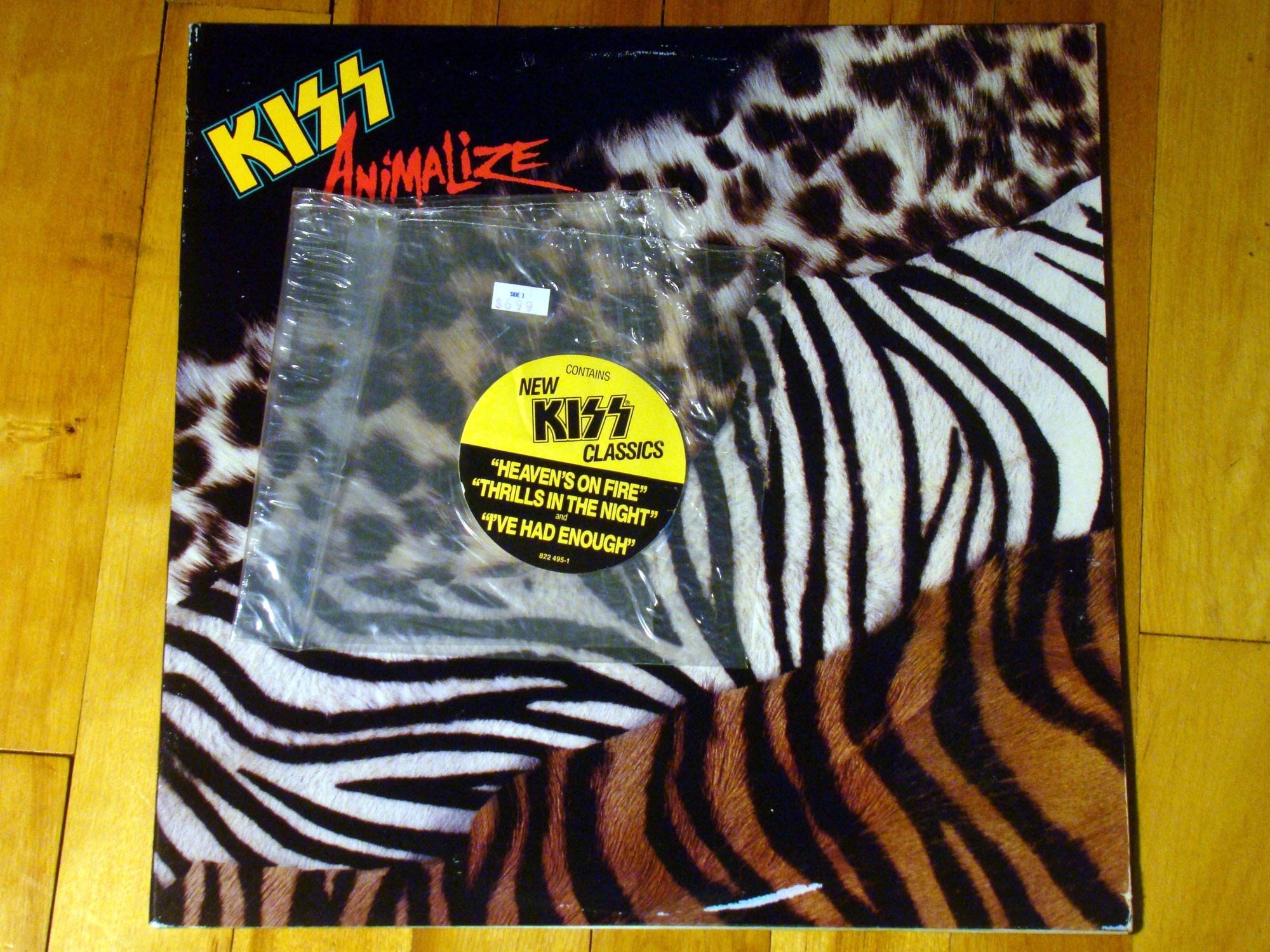This image showcases a worn album cover of KISS's **"Animalize"**, lying on a light-colored wooden floor. The album cover features the KISS logo in yellow, with its distinctive lightning bolt-shaped 'S's, positioned diagonally in the top left corner. Below the KISS logo, in bold red, the title "ANIMALIZE" is emblazoned in a dynamic, wild font. The design of the cover is split into several diagonal stripes, each representing a different animal print: starting with a cheetah print, followed by a white and black zebra print, and concluding with a tiger print at the bottom. 

Overlaying the album cover is a piece of square plastic, approximately four inches by four inches or slightly larger, holding a prominent circular sticker. This sticker is bisected into a yellow upper half and a black lower half. The yellow portion contains black letters stating **"NEW KISS CLASSICS,"** while the black section has yellow lettering listing the hit tracks "HEAVENS ON FIRE," "THRILLS IN THE NIGHT," and "I'VE HAD ENOUGH." The corners of the album cover are visibly scuffed, indicating wear and tear from use. This detailed composition highlights the distinct and nostalgic characteristics of the **KISS "Animalize"** album cover, enhanced by the overlaying sticker that denotes its classic tracks.